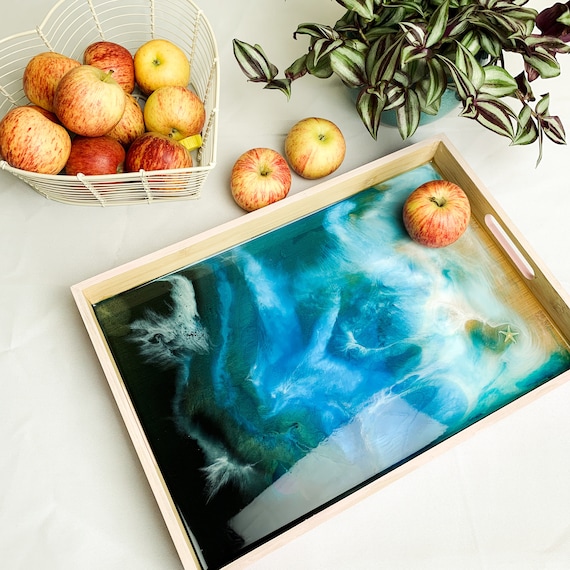The image features two distinct trays of apples placed on a white surface. At the top left, there's a light yellow, heart-shaped metal basket containing several apples with vibrant red and yellow-orange hues. In the center, there is a rectangular wooden tray, which appears to be made of bamboo, featuring handles on both ends for easy carrying. This tray contains a single apple, and showcases an abstract mat with green, blue, and white patterns that resemble an underwater scene with waves, possibly starfish. Between these trays, two additional apples are placed directly on the white surface. Near the top right corner of the image, part of a green plant can be seen, its leaves showcasing a gradient from light to dark, possibly a variety known as a praying mantis plant. The overall composition of objects on the white table emphasizes the colorful contrast of the apples and decorative elements.